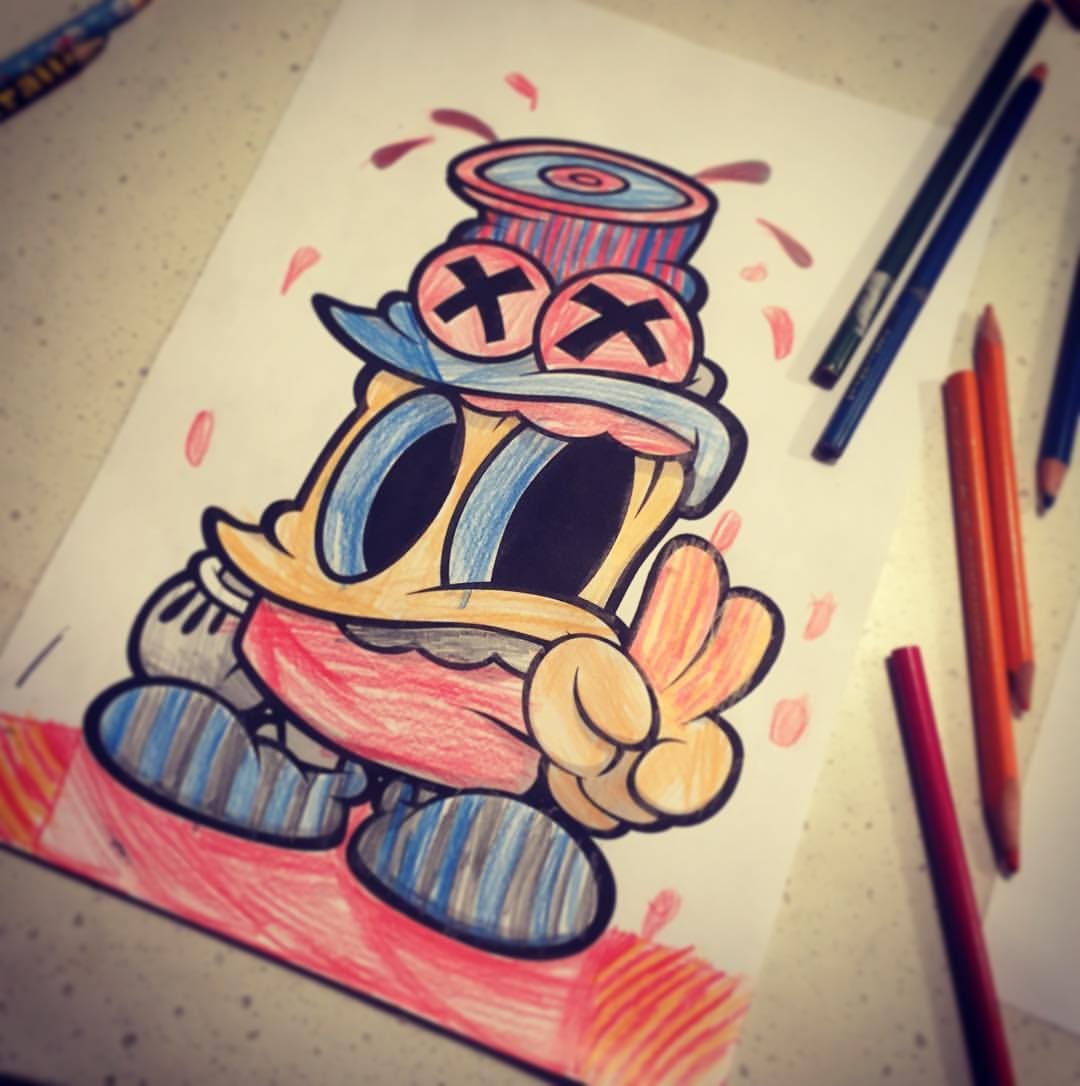The image is a square photo of a colored pencil drawing, set against a white granite-like countertop. The drawing appears slightly skewed, angled approximately 45 degrees to the right. Assorted colored pencils lie beside the drawing, suggesting they were used to complete it. The picture itself is on an A4 sheet of white paper and depicts a cartoonish, child-colored character. 

This peculiar character features a large head with two immense black eyes rimmed in blue, giving the impression of hollow sockets. Its face bears no discernible mouth or nose, though there is a prominent red area beneath the eyes which could be interpreted as the mouth or part of the body. The character sports a peculiar hat adorned with blue and red vertical stripes and topped with a red ring and a blue circle. Two orb-like decorations with black Xs sit atop the hat's brim, from which red drops appear to spill down.

The character's right hand is a white-gloved fist, while its left hand, also gloved, shows a peace sign with three fingers and a thumb. It has short, rounded legs with shoes featuring blue and black vertical stripes. Standing on a red platform or puddle, the character is surrounded by additional red and orange accents, perhaps indicating spilled liquid or a stylistic ground.

Overall, the image blends whimsical and eerie elements, highlighted by the colorful yet chaotic details of the child’s artistic efforts.